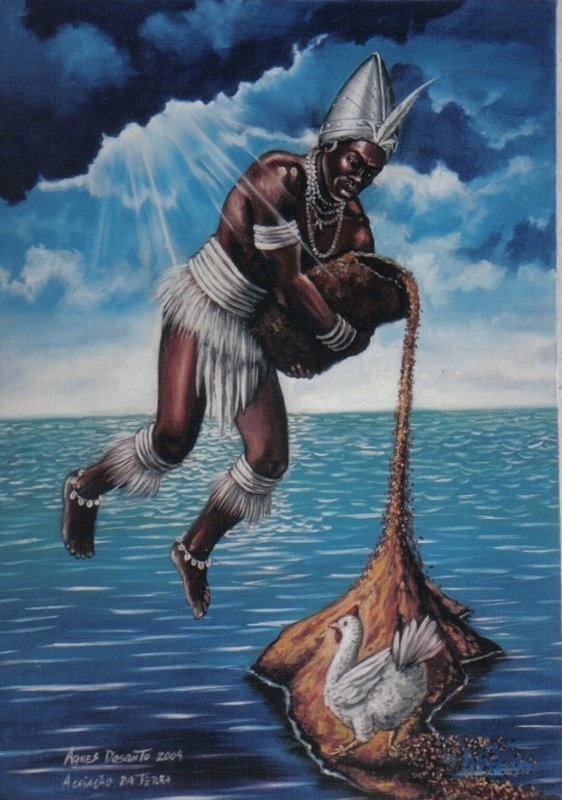This illustration, potentially a print or painting inspired by a mythological story, depicts a dark-skinned man hovering mid-air over the ocean. He wears an elaborate silver conical hat adorned with a feather, multiple silver chain necklaces, and chain bangles on his upper arms and wrists. His attire includes a feathered loincloth and bands with additional feathering around his lower legs, concluding with ankle bracelets. The man is muscular and shirtless, facing the right side of the image. He pours a substance from a burlap or canvas bag, creating an island-like mound in the water below him. A white chicken is actively scratching at this newly formed pile. The backdrop features a cloudy sky with sunbeams breaking through from the upper left corner. The artist, inscribed as Agnes DeSanto, 2004, is signed in the bottom left-hand corner of the image.